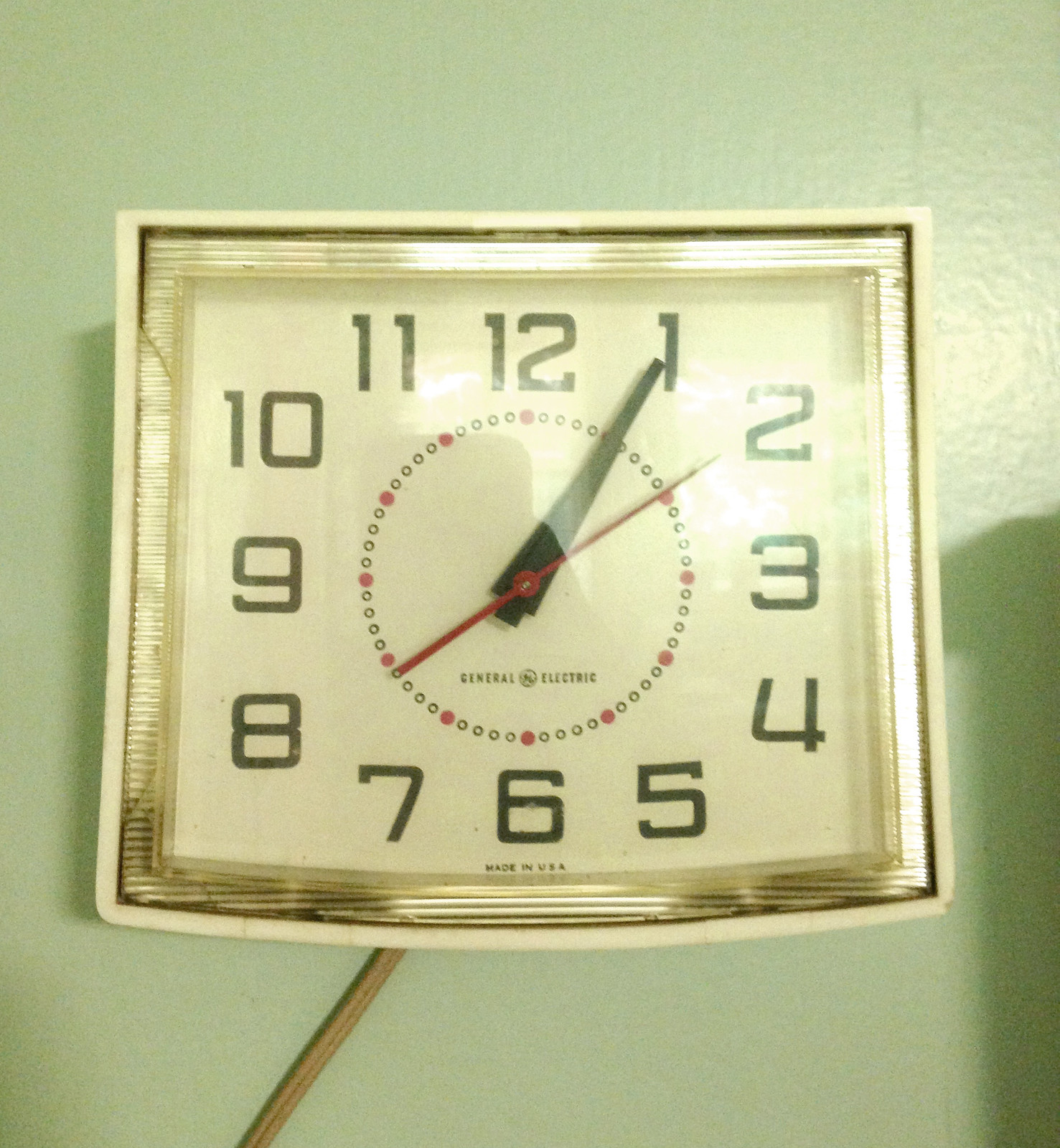This photograph captures a rectangular clock with a slightly rounded bottom, mounted on a soft, pastel lime-green wall, with a gray cord extending towards the lower left side of the image. The clock features a white-tan outer frame, while the face of the clock is white, encircled by a square gold section. Bold black numbers mark each hour, organized into four vertical and horizontal sets. The clock’s hands include a black hour and minute hand, and a long, thin, red second hand, currently pointing at 10 seconds past 1:05. Minute markers consist of alternating red filled circles and black empty circles. Below the six, the inscription "Made in USA" is visible, while the clock's center bears the manufacturer’s name, "General Electric."